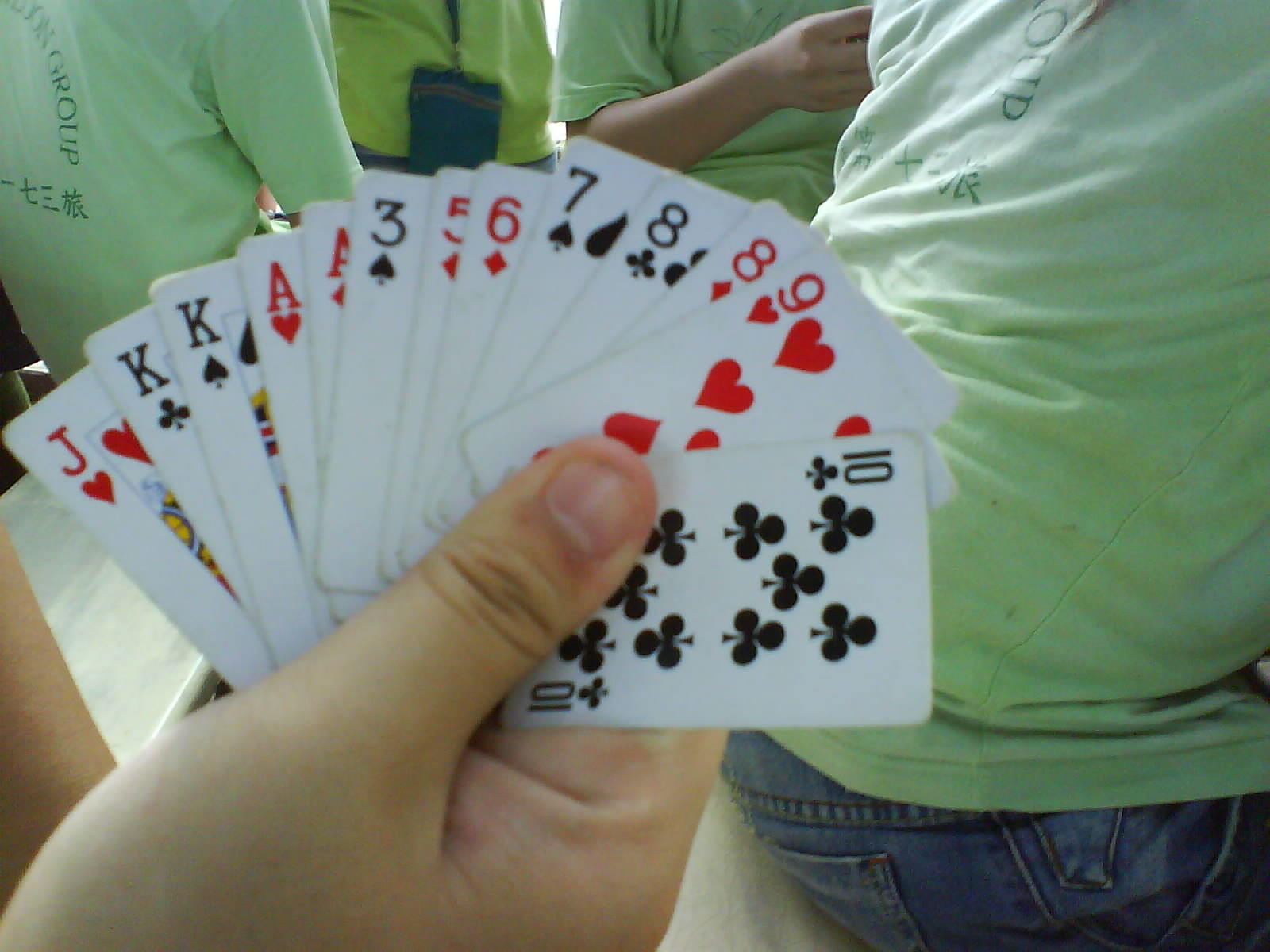The photograph features an individual firmly holding a fanned-out hand of 13 miniature playing cards in their right hand. The cards, listed from left to right, include the Jack of Hearts, King of Clubs, King of Spades, Ace of Hearts, Ace of Diamonds, Three of Spades, Five of Diamonds, Six of Diamonds, Seven of Spades, Eight of Clubs, Eight of Diamonds, Nine of Hearts, and Ten of Clubs. The cards are notably smaller than a standard deck, each card no longer than the individual's thumb, confirming their miniature size rather than an optical illusion.

In the background, there is a group of people wearing light green short-sleeved t-shirts. The word "GROUP" is visible on the back of several t-shirts, which also feature Oriental writing that appears to be in Japanese, Korean, or Chinese. Further in the background, an individual in a deeper greenish-yellow t-shirt is visible. This individual wears a lanyard with an ID card or document holder hanging down to their belt. Overall, the scene offers a candid glimpse into a social setting involving a card game, with culturally diverse elements and an organized group atmosphere.